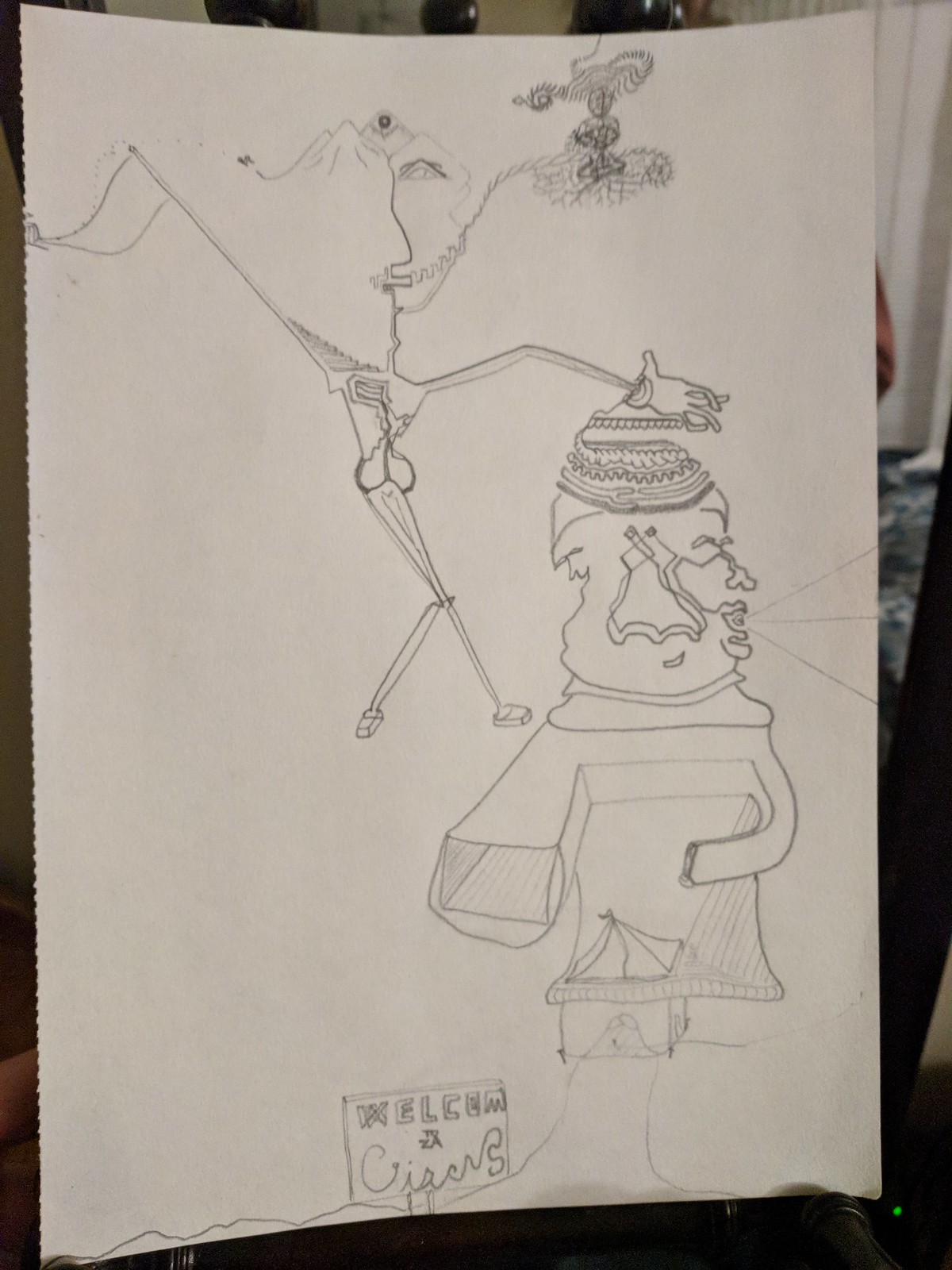This photo captures a detailed and imaginative piece of artwork drawn on white paper. The drawing, in pencil, incorporates a variety of characters and elements, creating a whimsical and intricate scene. At the very bottom of the artwork, there's a sign that reads "Welcome" and possibly "Circus." Above the sign, the scene unfolds into a series of fascinating characters.

One character resembles a tent or house that you might walk into, blending elements of architecture with anthropomorphic features. Another prominent figure near the top of the drawing looks like human bones, with steps leading off its shoulder that transition into various surreal elements. 

Among these elements is a flag and a half-face that creatively morphs into a mountain range. This half-face appears to be smoking a cigarette, with the smoke intriguingly depicted as a zipper. The smoke trails off towards the upper right part of the paper, culminating in what resembles a genie bottle. The artist has infused the piece with a blend of surreal and imaginative features, showcasing their creativity through this captivating drawing.